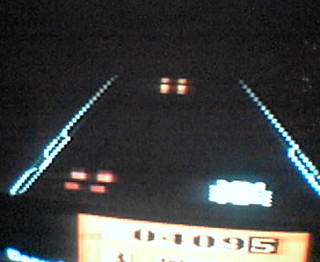The image appears to be a blurry and blown-out screenshot from a video game. The scene is predominantly dark, with the black background making the bright elements stand out. The composition suggests a one-point perspective reminiscent of a road or runway extending towards the horizon, with lines converging from both the left and right sides of the screen. Four small reddish-orange lights are positioned near the top and towards the back, possibly resembling fireballs or runway lights. In the foreground, there are additional four bright reddish-orange lights arranged in a grid pattern. On the bottom of the image, a partially visible electronic screen displays a rectangle with an orange background and black text reading "0409," alongside another black rectangle containing the number "5" in white. The right side of the image features a blown-out, indiscernible cluster of white or light blue lights. The entire image is slightly wider than it is tall, and the overall visual quality is very blurry and blown out, making precise details difficult to discern.